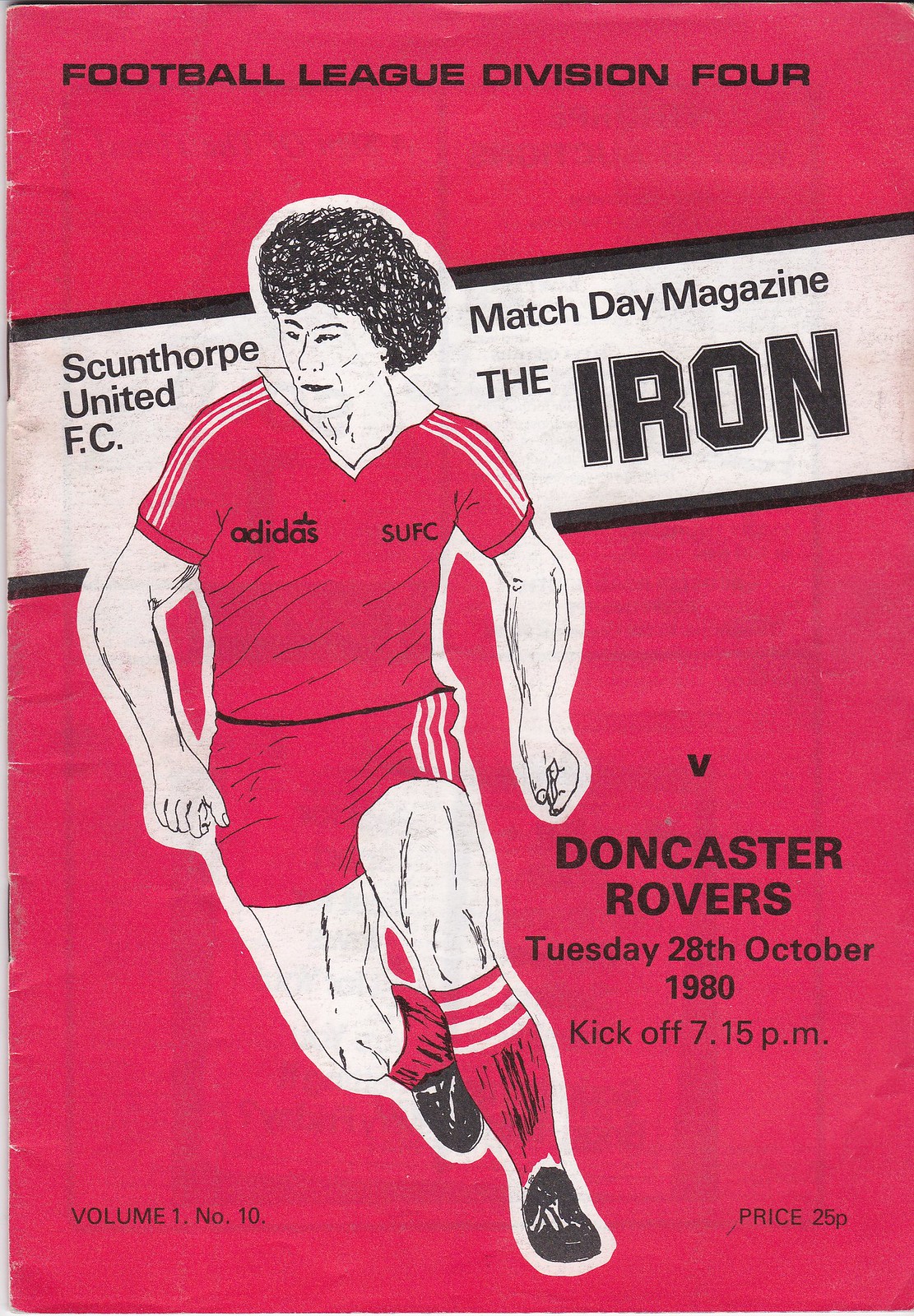The image features the cover of a Match Day Magazine for a Football League Division IV game, dating back to Tuesday, 28th October 1980, with a kickoff time at 7:15 p.m. The predominantly red cover is adorned with a detailed sketch of a football (soccer) player in motion, running towards the right. The player is outfitted in all-red Adidas attire, including a t-shirt, shorts, knee-high socks, and black shoes, and sports a black afro hairstyle. The heading reads "Football League Division IV", and beneath it is the text "Scunthorpe United FC, Match Day Magazine, The Iron vs. Doncaster Rovers." Additional details include the price of the magazine (25p), the volume (Volume 1, Number 10), and a banner featuring the same heading, angled behind the player. The magazine predominantly uses red, black, and white colors.